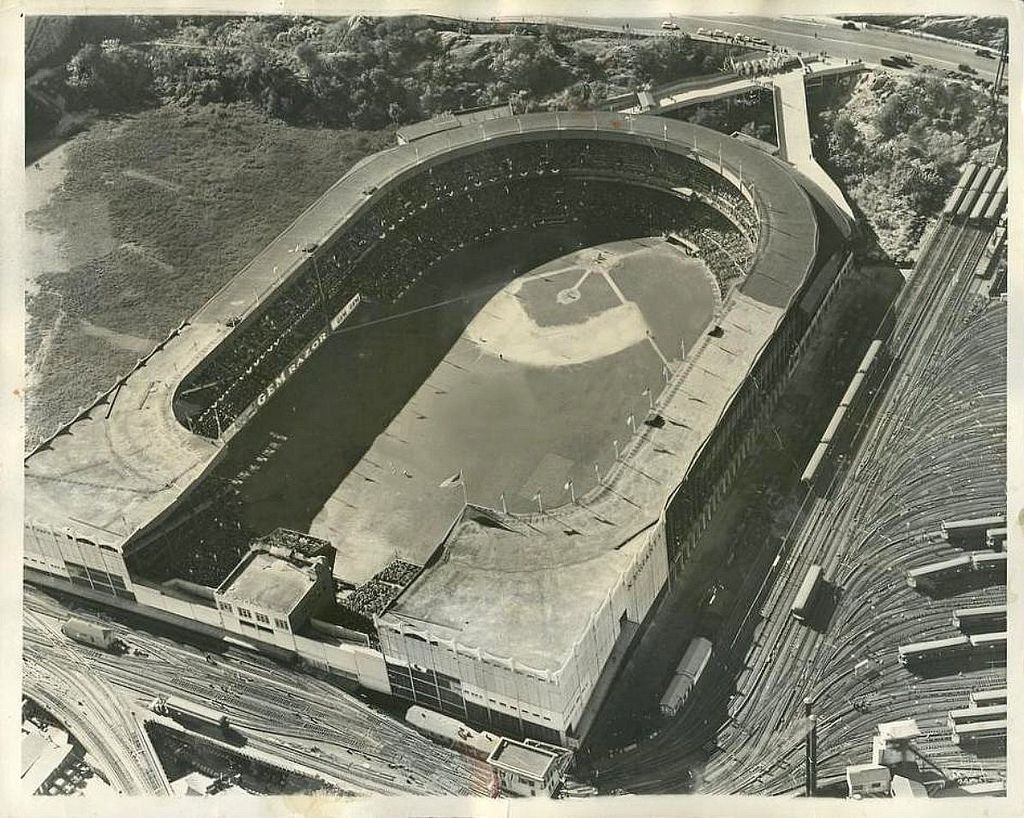This is a black and white aerial photograph of an old baseball stadium, likely one of the earliest built. The stadium has an ovular shape that meets with a rectangular section at the bottom, forming a horseshoe-like structure. The stands appear to be packed with spectators, though they seem tiny due to the high vantage point from which the photo was taken. On the field, players can be seen in their positions, despite the initial impression of emptiness. The area surrounding the stadium features a mix of greenery, highways, access roads, and extensive train tracks laden with train cars, especially prominent on the right side extending towards the front. A banner along the side of the stadium reads "Gemraiser" or possibly "Gem Razor," subtly illuminated from the left side of the photograph, casting shadows. The overall scene captures the bustling, historical essence of early baseball.